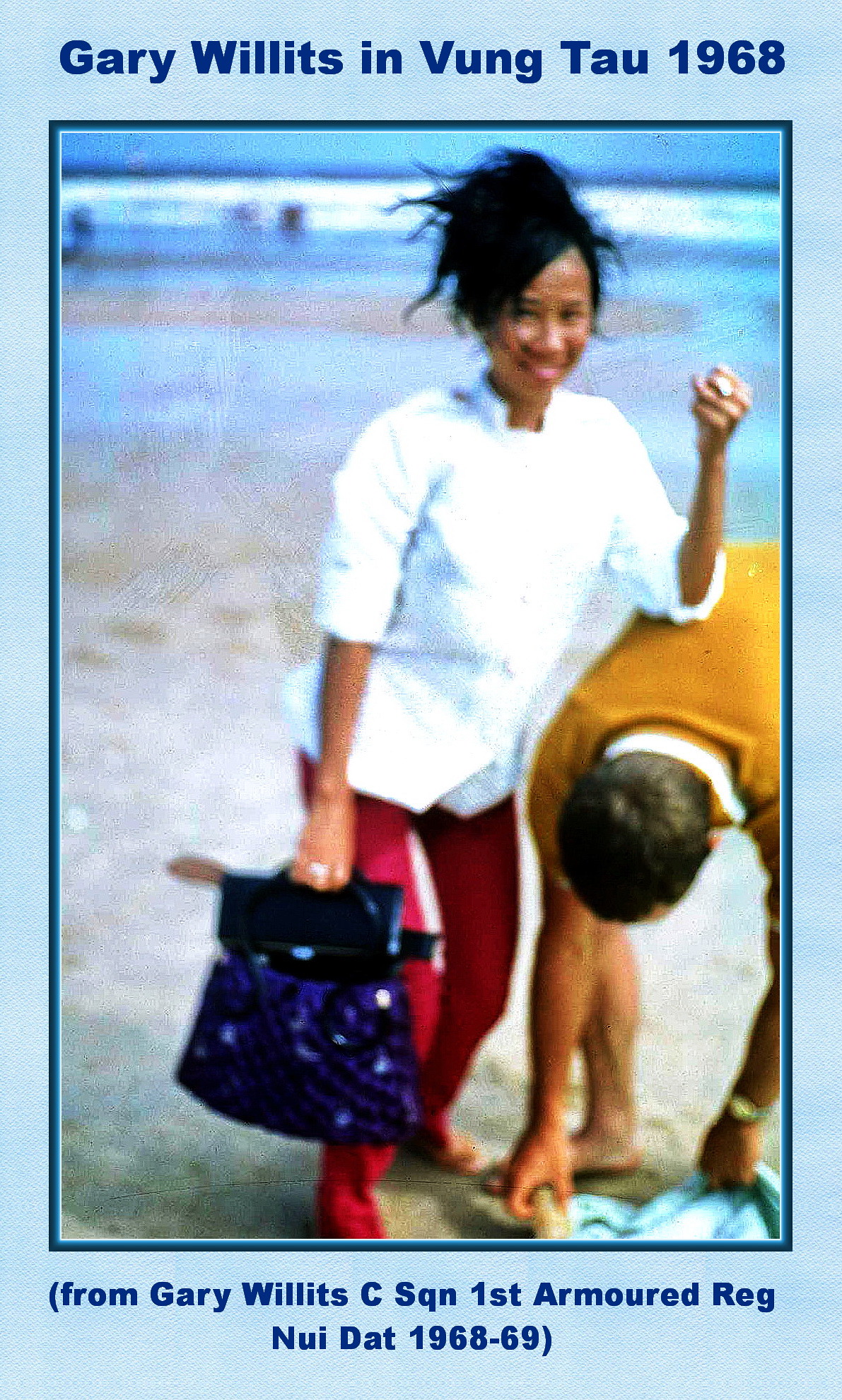The image, bordered in blue, is captioned at the top with the text "Gary Willits in Vung Tau, 1968." Below, additional text reads: "Gary Willits, C.S.Q.N., First Armored Reg, N.U.I.D., 1968-69." The scene depicts a sunny beach in Vung Tau, Vietnam, against the backdrop of a clear blue sky and crashing waves. At the center is a young woman with brown or black hair styled in an updo, wearing a white long-sleeved shirt with the sleeves rolled up, red pants, and a ring on her finger. She holds a purple purse and stands beside a man who is kneeling down, wearing an orange or yellow shirt. The setting suggests a moment of leisure amidst the tumultuous times of the Vietnam War.